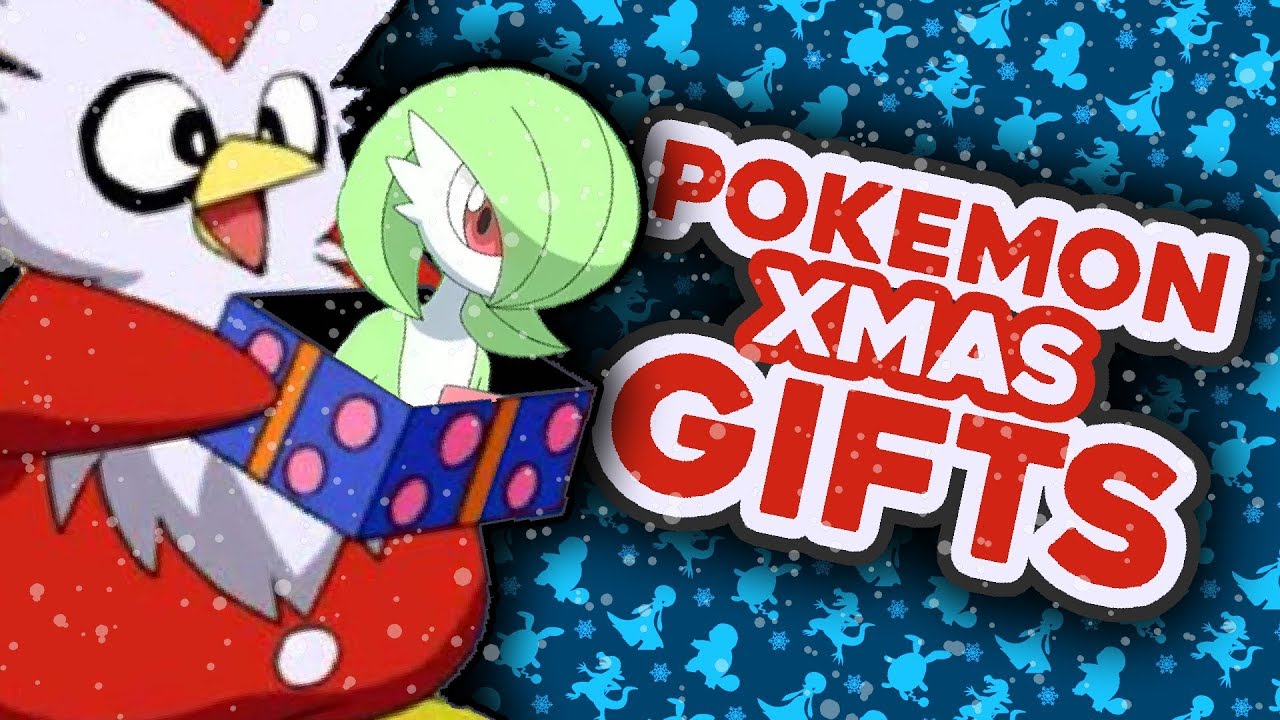The image depicts a festive scene set against a blue background, featuring two distinct Pokemon characters. The primary character is Delibird, a bird-like Pokemon with red feathers and a white torso. Delibird has a yellow beak and is holding a present. The gift is a blue box adorned with pink circles and a single orange stripe running down the center of each side.

Beside Delibird is a second Pokemon, Galarian Slowking. This creature has striking green hair that is slicked back over his face, revealing one red eye partially obscured by the hair. The green plumage starts at the base of his beak, which is also green.

The image includes text promoting a "Pokemon Christmas XMAS" theme. The word "Pokemon" appears in red on a white background, while "Christmas" is written in white on a red background. The word "Gifts" is presented in red on a white background.